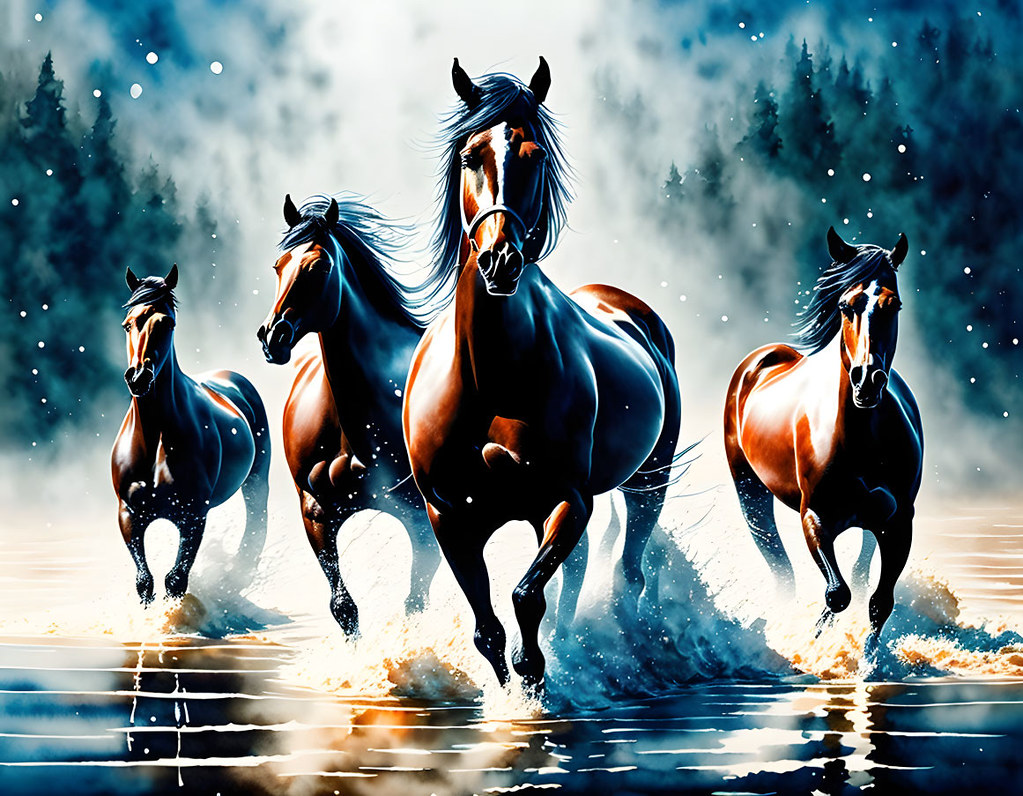This captivating painting portrays four brown horses galloping through water towards the viewer, each seemingly racing against the misty backdrop of towering evergreens. Their wet coats gleam under the light, with patches of white scattered across them, conveying their sleek movement. The lead horse—a large, powerful stallion—charges forward, its mane and ears swept back by the speed, followed by a slightly smaller mare and two even smaller mares on either side, possibly indicating varying ages or simply differences in perspective. The water beneath their powerful strides is alive with splashes, ripples, and foaming waves, adding to the dynamic energy of the scene. The background, a surreal mix of blue-gray hues and fog, interspersed with subtle white spots that might suggest snowflakes or sunlight breaking through the trees, enhances the dramatic tension, hinting at an elusive story behind the horses' urgent dash through the shimmering water.